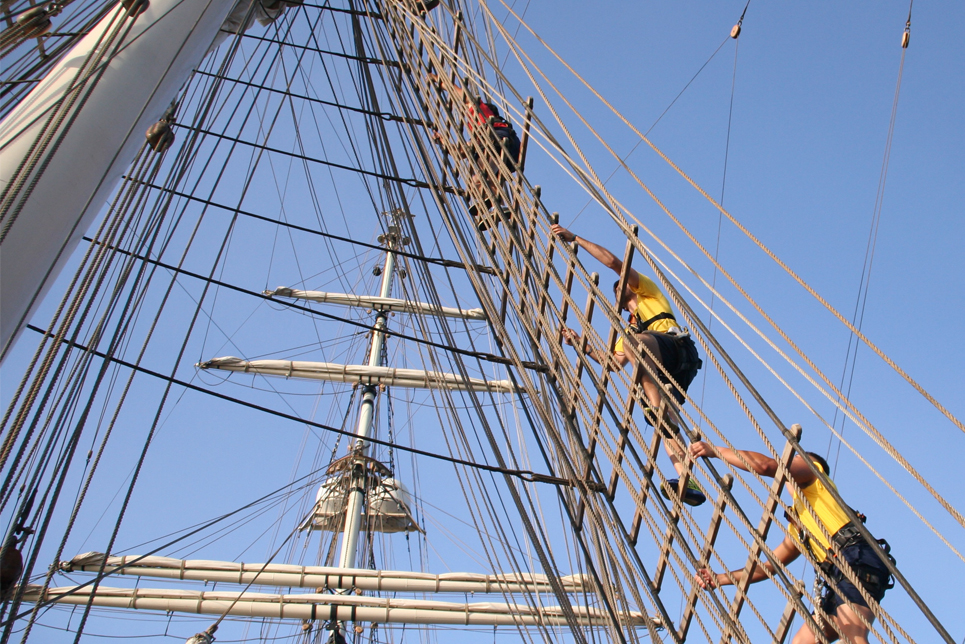The photograph captures a striking scene aboard an old-fashioned sailing ship, reminiscent of the historic Mayflower. The viewer's perspective is from the deck, looking straight up at the towering main masts. The clear blue sky provides a vivid backdrop to the image, contrasted by the white pole at the center. The ship is at sea, indicated by the setting and the workers scaling the sides.

In the foreground, three individuals climb a brownish ladder angled up the side of the ship. They appear to be secured with small ropes for safety. The climbers include one person in a red shirt and black shorts at the top, and two others in yellow shirts and dark-colored shorts following behind. Their colorful attire stands out against the intricacies of the ship's structure.

The ship's masts rise majestically towards the sky, with the rigging—dark cables, pulleys, and ropes—intricately detailed and crisscrossing the scene. Four large, white sails are tied up and not unfurled, with what appears to be a crow's nest situated between them. The abundance of lines and rigging accentuates the complexity of the vessel, hinting at the age-old maritime traditions still in practice. The bright, cloudless day enhances the visibility of every minute detail, from the subtle hardware securing the masts to the determination of the workers scaling the heights.